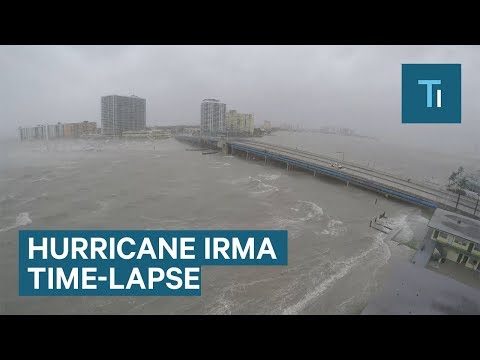This photograph, captured from an elevated perspective during Hurricane Irma, depicts a stormy, fog-obscured scene dominated by a large, grayish water body with turbulent waves and visible white bubbles indicating violent swirling. Prominently crossing the middle of the water is a bridge, with several tall buildings lining the shore in the background, particularly larger ones on the front shoreline and smaller ones towards the bottom right. The entire image is cast in a muted gray color theme, echoing the overcast, light gray sky. Notably, in the top right corner, there is a square logo with the letters "TI," and at the bottom left corner, white, all-capital text in a sans-serif font reads "HURRICANE IRMA TIME LAPSE," set against a blue background. The photograph is bordered at the top and bottom by horizontal black strips, framing the intense depiction of the flood caused by the hurricane.